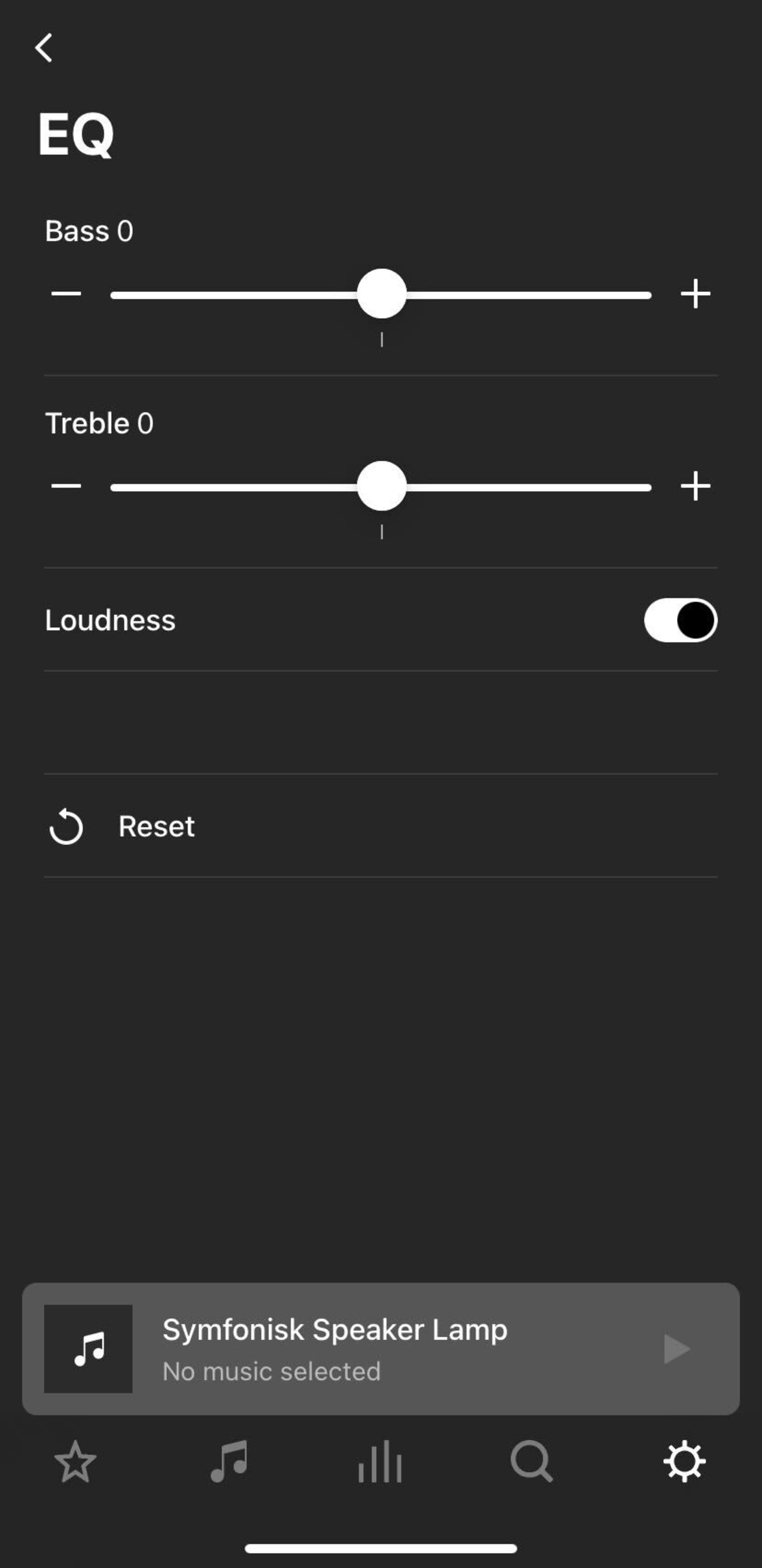This is a detailed screenshot from a mobile phone displaying an audio settings interface with a charcoal black background. At the top of the image, there is a small, left-pointing arrow indicating a back navigation option. Below this, the heading "EQ" is prominently displayed in bold white font. 

Underneath the "EQ" heading is the first control indicating "Bass" set at zero, accompanied by a horizontal white line slider with adjustable circular handles for increasing or decreasing the bass level. Directly below, the interface shows "Treble," also set at zero, with a similar adjustable slider provided to modify the treble levels. 

The next control in the sequence is “Loudness,” which has a switch toggled to the "on" position, suggesting it has been activated. Beneath the loudness control is the "Reset" option written in white font, paired with a white refresh icon to its left, which likely allows the user to revert settings to their default values.

At the very bottom of the screen, a gray rectangular section displays the text "Symphonesque Speaker Lamp, no music selected," indicating that no music is currently playing. To the left of this text is a dark black square containing a white musical note icon, indicating a link to the music library or controls.

This comprehensive screenshot details the various audio customization options available on the mobile phone’s interface.